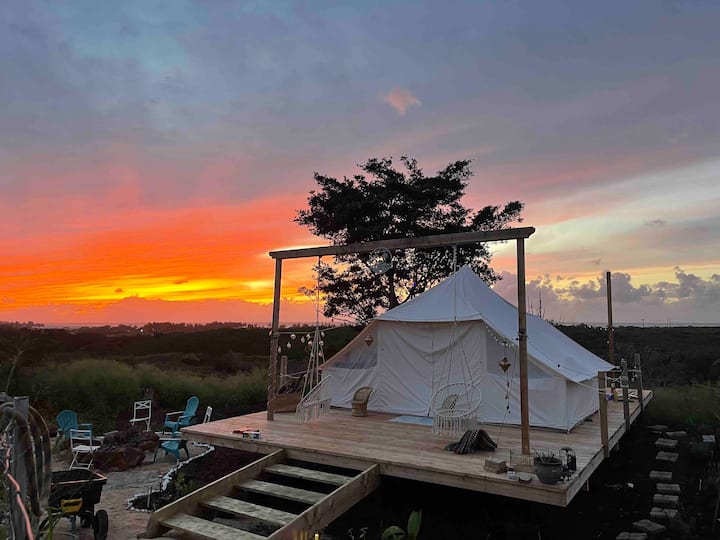The image depicts a serene outdoor scene at sunset, showcasing a large white tent perched on an elevated wooden platform, accessible via a wooden ladder or bridge. This unfinished light brown wooden deck lacks railings and appears recently constructed. The tent, tethered to surrounding wooden posts to prevent it from being displaced by the wind, has a spacious appearance.

In front of the tent stands a distinct wooden archway from which hang two basket swings. A blanket is casually laid next to the foremost swing, enhancing the cozy atmosphere. Various chairs in shades of turquoise, blue, and white are scattered around the area, including some placed near a fire pit and on the lower level of the decking. The platform is bordered with planters and bricks, adding to the rustic charm.

The backdrop features lush greenery with grass, shrubs, and possibly distant trees or buildings. The stunning sky transitions from a fiery yellow-orange near the horizon to a cooler blue as it stretches away from the sunset, with a sprinkle of clouds reflecting the twilight hues. This idyllic setup appears to be a perfect spot for relaxation and gathering, set against the enchanting canvas of a setting sun.